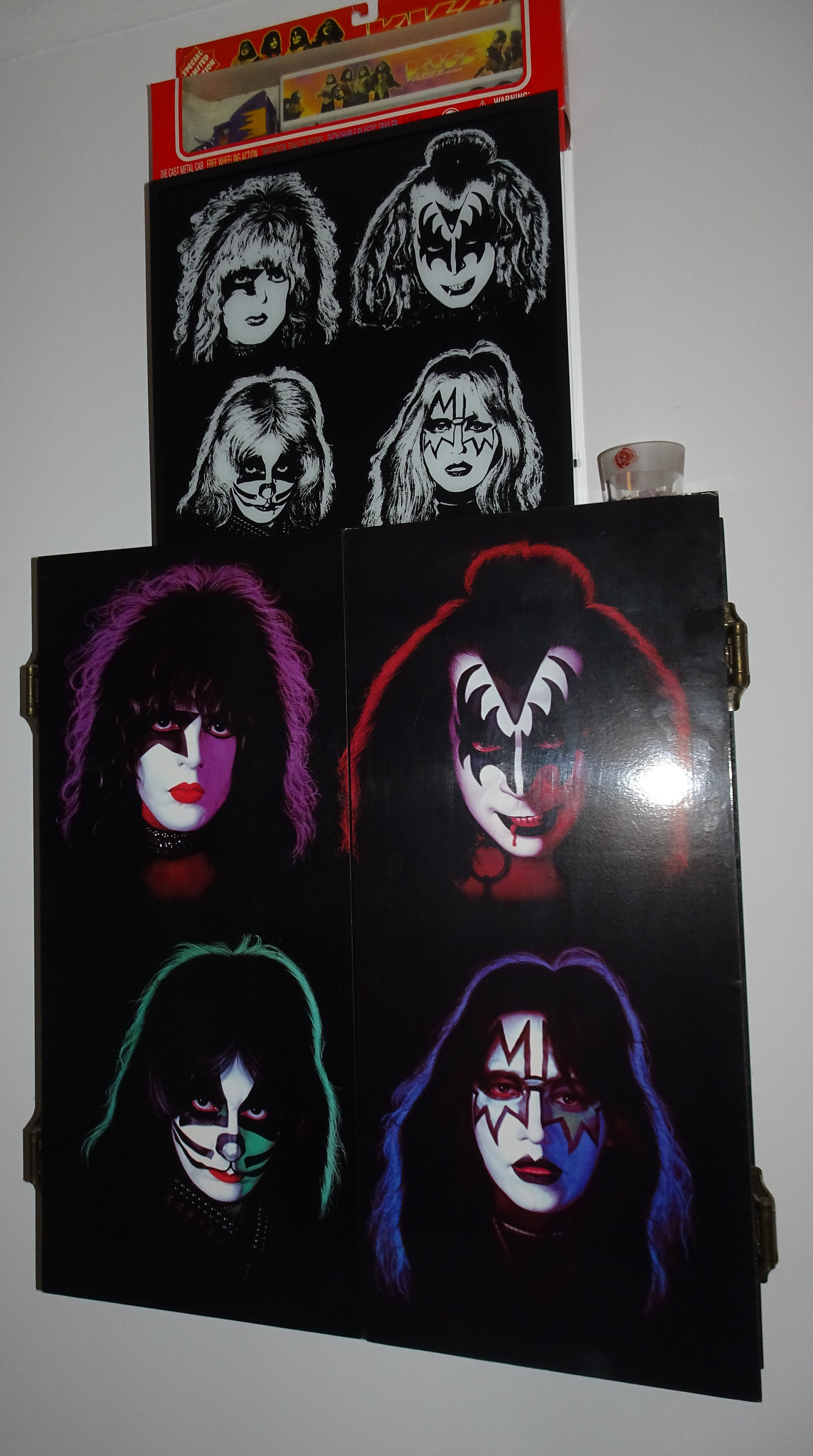This photograph captures a bedroom wall adorned with two posters and a box of figurines, all celebrating the iconic rock band KISS, famous for their demonic clown makeup and theatrical performances in the late 1970s. The wall itself is white, providing a stark backdrop for the vivid imagery. 

The top poster is a black-and-white image of the four band members' faces, each meticulously painted with their signature makeup, set against a black background. Below this, there is a larger, color version of the same image. This colored poster dramatically highlights the band members: one is surrounded by a pink glow with fluffy hair and a black star over the left eye; another sports fluffy hair in a bun, with black wing-like designs around the eyes and a triangle extending from the forehead to the nose. The third member has a greenish glow, rectangles around the eyes, and stripes on the cheeks and nose, while the fourth is enveloped in a purple afterglow, with pinkish-white wings painted around the eyes.

Above these posters sits a box that appears to contain KISS figurines, adding a three-dimensional element to the display. Both posters are designed to resemble shutters, complete with hinges on the sides, intensifying the rock-and-roll aesthetic. The meticulous details in the band members' makeup and the dramatic use of color versus black-and-white imagery capture the electric essence of KISS, resonating with the shared visual language of their fans.